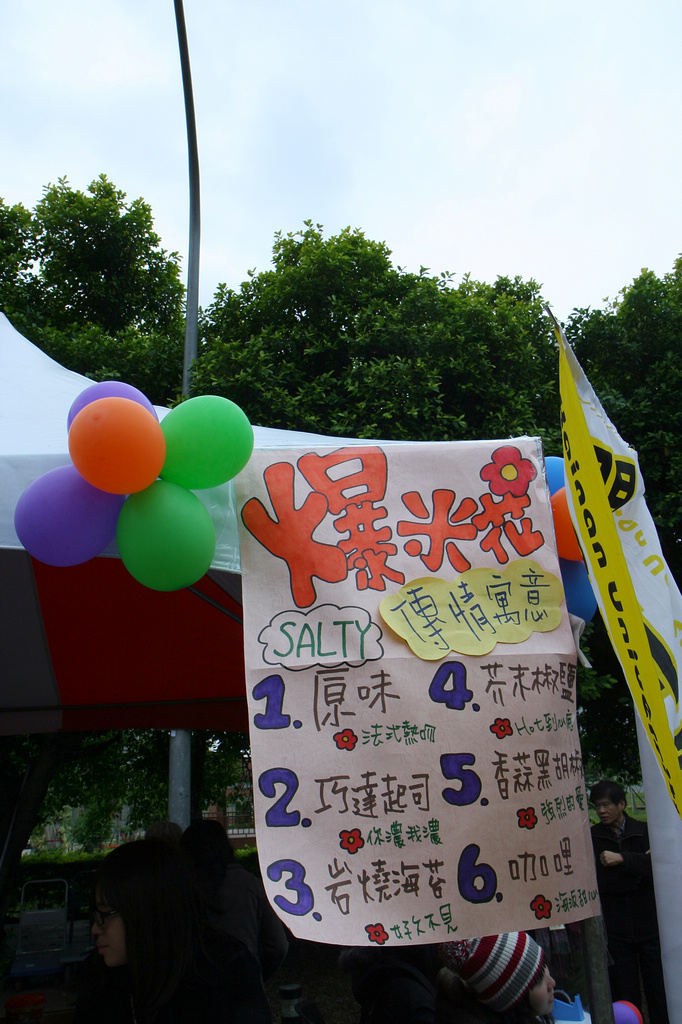This vibrant photograph captures the lively atmosphere of an outdoor celebration, likely a party or festival. Dominating the center of the image is a tent adorned with an array of colorful balloons in hues of orange, green, purple, red, yellow, and blue. A banner hangs prominently on the tent, featuring text in an East Asian script, with the word "salty" standing out in English. The setting appears to be under a partly cloudy sky, evident from the visible clouds overhead, with tall trees providing a lush green backdrop. In the foreground, several people are seen engaging with activities around the tent, suggesting a lively gathering. The image is bathed in daylight, highlighting the cheerful and festive mood of the scene.